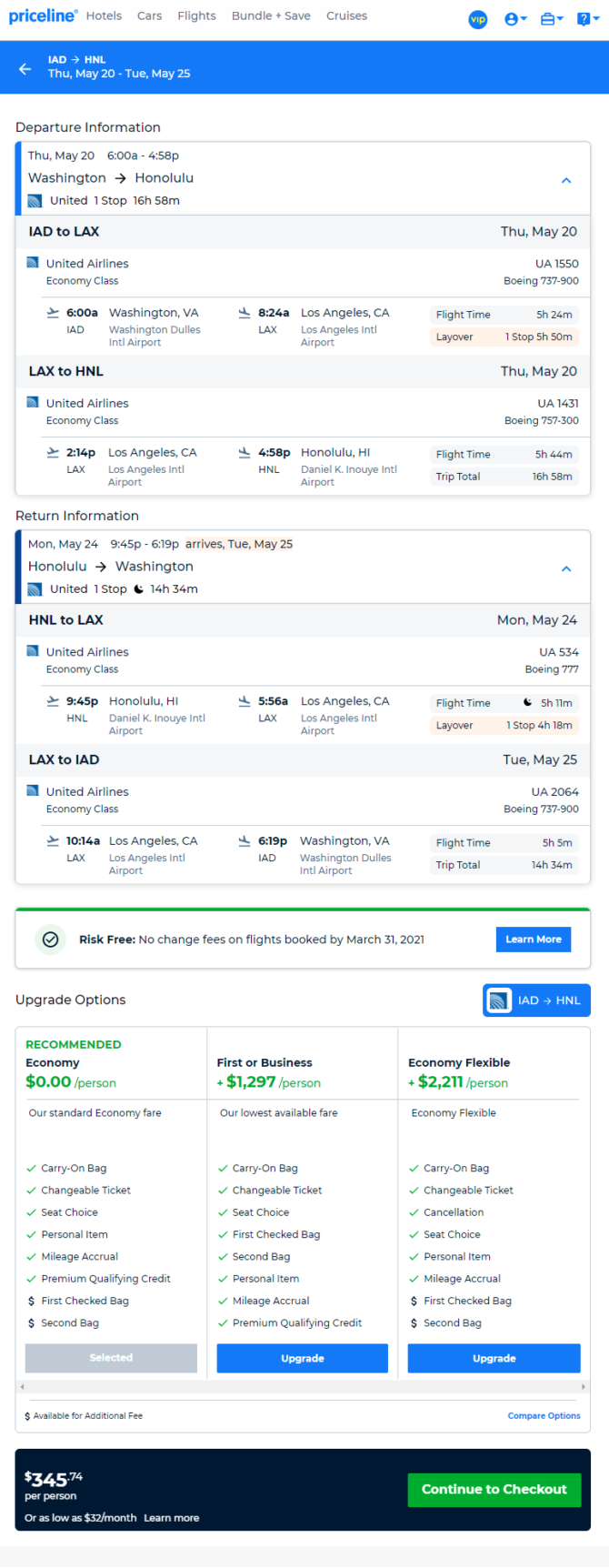The image captures a screenshot from the Priceline website, showcasing travel itinerary details for a trip from Washington to Honolulu. At the very top, against a blue background, the Priceline logo is prominently displayed. Below the logo, there are dropdown menus labeled "Hotels," "Cars," "Flights," "Bundle and Save," and "Cruises." A VIP section and several icons are also visible on the top bar.

A blue rectangle spans the top of the itinerary section, listing the travel dates as "Thursday, May 20th to Tuesday, May 25th." Beneath this, the heading "Departure Information" is displayed, with specific details for the outbound flight. The departure is scheduled for Thursday, May 20th, from 6 a.m. to 4:58 p.m., traveling from Washington (IAD) to Honolulu, with a single stopover. The flight is operated by United Airlines, with a total duration of 16 hours and 58 minutes. The itinerary further specifies the first leg of the journey from Washington Dulles International Airport (IAD) to Los Angeles International Airport (LAX), including a note about a five-hour layover.

In the same section, the return flight information is also provided, detailing the journey from LAX back to IAD. 

At the bottom of the layout, three rectangular options are presented, highlighting different travel classes: "Recommended" economy, first or business class, and economy flexible. Additionally, there’s a box asserting a "Risk-free, no charge fees on anything" policy, emphasizing flexibility for travelers.